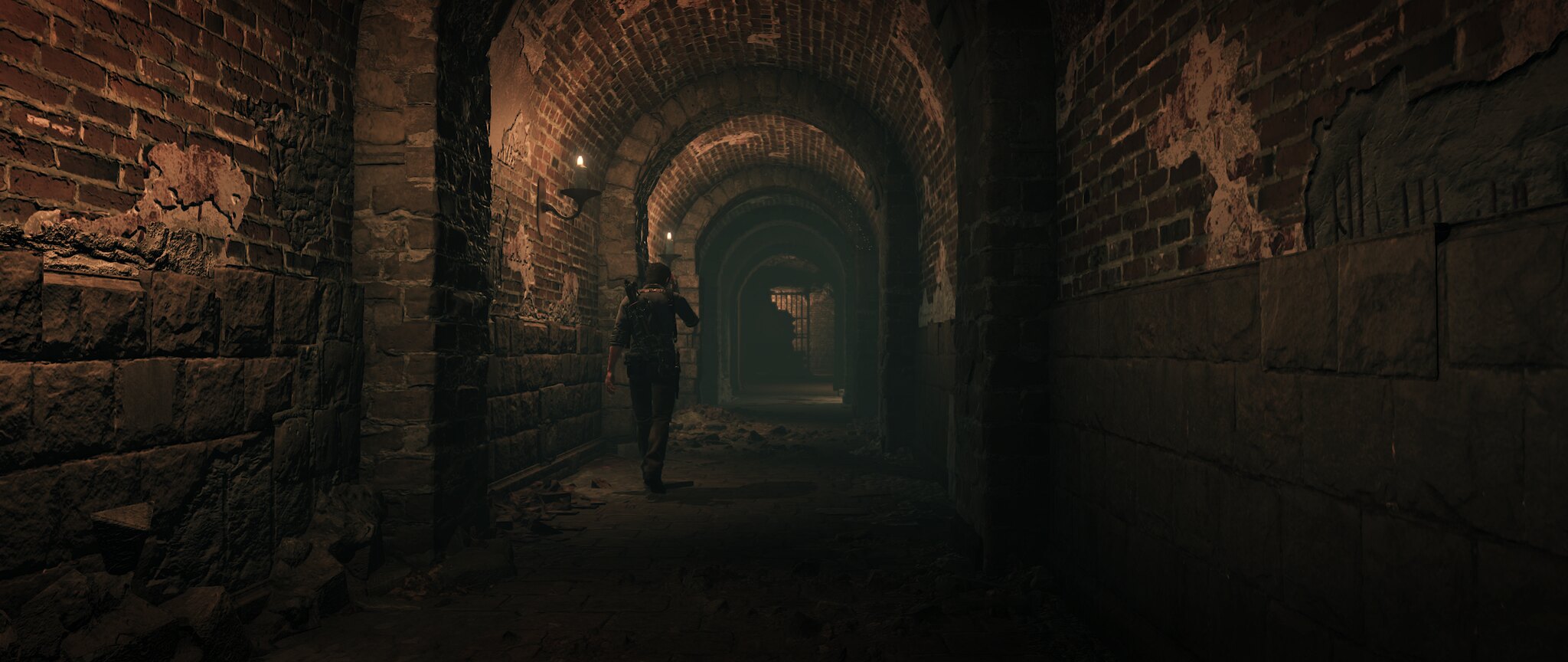The image appears to be computer-generated, depicting a dimly lit, arched tunnel that is evocative of a video game setting. The tunnel is framed by decrepit brick walls on both sides, with sections appearing broken and ragged. The lower part of the walls transitions into stone, adding to the ancient and worn ambiance. As the tunnel extends forward, you notice a series of repeating archways that enhance the sense of depth and enclosure.

A character, seen from behind, is walking down the tunnel towards an end that features a barred doorway, almost resembling a cage. The character is dressed in pants and a shirt with sleeves either pulled up to or ending at the elbows. Their left arm hangs by their side as they make their way forward.

Lighting in the tunnel is sparse, contributing to the moody atmosphere. Candles affixed to the walls in sconces provide the minimal illumination, casting flickering shadows on the brick and stone surfaces. At the end of the tunnel, in the dimly lit barred doorway, there appears to be a mysterious, hulking silhouette, adding an element of foreboding to the scene.